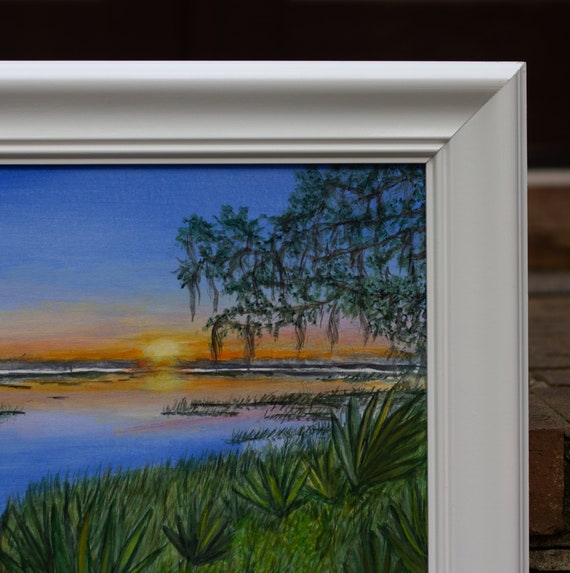A detailed zoomed-in image captures the upper right-hand corner of a white, slightly concave, and beveled picture frame. The painting within the frame depicts a captivating waterscape with green grass and tall plants at the forefront. The scene reveals a serene body of blue water dotted with patches of marsh grasses and bogs, extending towards a distant horizon. There, gentle waves crest beneath an enchanting sunset, casting hues of orange and yellow across the sky and water, while remnants of blue sky suggest the dawn of the day. A large tree with drooping branches is visible, adding to the immersive, almost swamp-like ambiance of the scene. The painting appears to be propped against a black-background surface, possibly a brick patio, invoking an intimate and rustic charm.